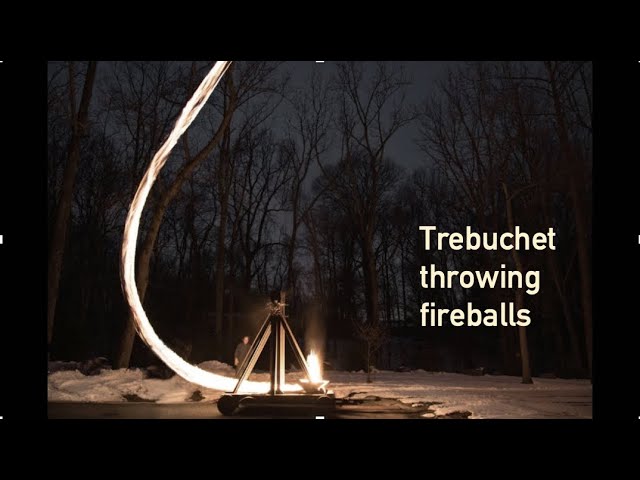This nighttime photograph, bordered in black, captures a snowy forest scene under a dark, greyish-blue sky. The leafless, silhouetted trees frame a wooden trebuchet with a triangular structure, stationed centrally. A man, indistinct in details, stands behind the trebuchet. The ground beneath is blanketed in snow, adding to the wintry atmosphere.

The trebuchet appears to be in mid-action, launching a fireball. A vivid, curving arc of fire starts from the bottom of the trebuchet, rising upwards and to the left, forming a semi-circular trail reminiscent of the letter C. This bright arc illuminates the surrounding area, casting a warm glow over the snow.

Overlaying the bottom right of the image is white text that reads "trebuchet throwing fireballs," clearly identifying the scene. This detailed depiction emphasizes the stark contrast between the fiery motion and the serene, cold environment.